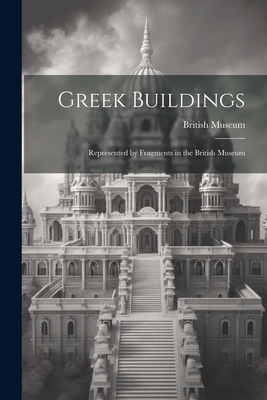This black and white vertical poster features a detailed image of a grand, white multi-story building, reminiscent of a museum or monumental architecture, prominently labeled "Greek Buildings" across the top, followed by "British Museum." The structure, surrounded by wide, cascading staircases similar to pyramid steps, is adorned with numerous windows and intricate carvings. The building's design includes a series of domes and columns, culminating in a large fluted dome at the summit, topped by multi-layered spires. Additional text beneath "British Museum" suggests a representation of fragments in the museum. The clouds in the background add to the majestic and historical ambiance of the image.